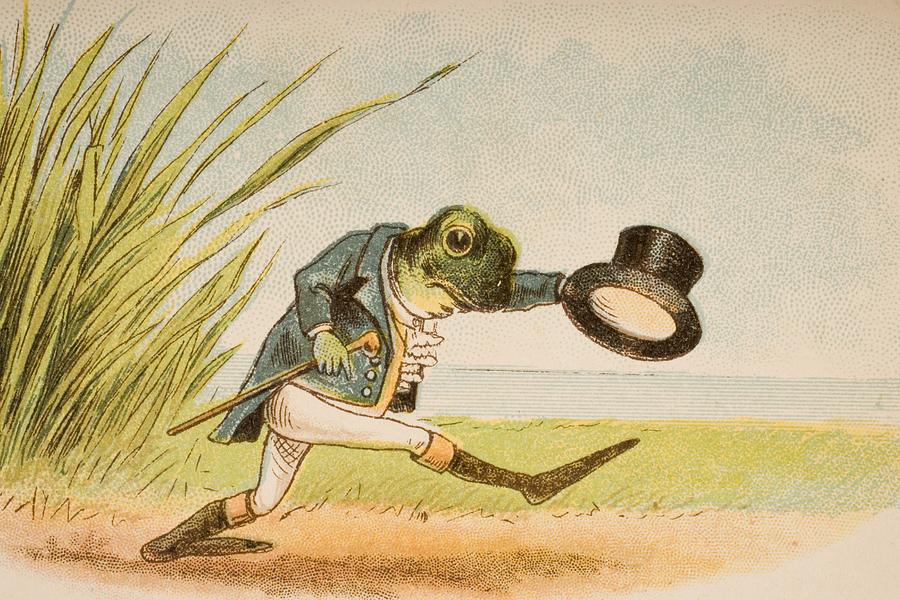The image depicts a whimsical illustration reminiscent of a children's book, featuring a frog that evokes characters from classic tales like "Frog and Toad." The frog, donning a sophisticated outfit, is dressed in a green or turquoise jacket, a frilly white shirt, and tight white pants that end in high black boots with cuffs around the knees. He sports a black top hat, which he holds ceremoniously in his outstretched left hand, and a straight cane in his right. The frog is taking long, confident strides along a dirt path, with one leg stretched out before him, almost as if he is dancing or taking a bow. His expression is neutral, though his large black eye seems to engage with the viewer. The background features a blend of soft, muted colors, possibly watercolor or pencil-like in texture. The scenery includes short grass and taller, swampy grasses that tower over the frog, against a backdrop of blue sky with hints of white clouds and water beneath it. The overall scene is charmingly detailed, capturing a moment of genteel animation in a serene, picturesque setting.